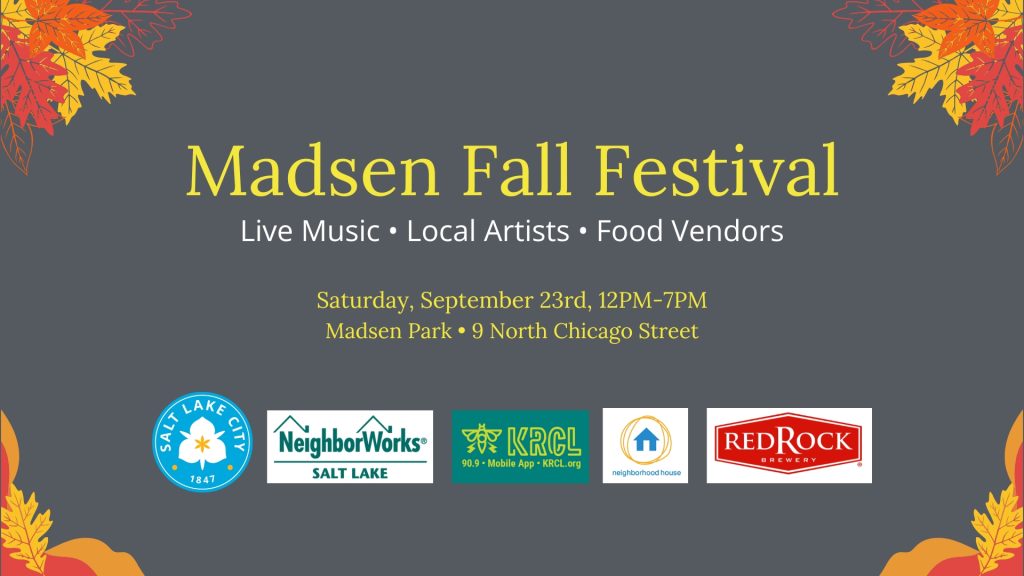The image is a digitally designed poster or flyer for the Madsen Fall Festival, prominently featuring fall-themed artwork. The poster's background is light gray, with artistically drawn autumn leaves—colored in shades of red, orange, and yellow—adorning each corner. In the center, bold yellow text announces the "Madsen Fall Festival," followed by white text detailing the event's offerings: "Live Music, Local Artists, Food Vendors." Additional yellow text below specifies the event's date, time, and location: "Saturday, September 23rd, 12 p.m. to 7 p.m., Madsen Park, 9 North Chicago Street."

The lower section of the poster includes five sponsor logos. From left to right, these logos are:
1. A light blue circle with a white flower, representing Salt Lake City.
2. A white rectangle with green text and two mountains, belonging to NeighborWorks Salt Lake.
3. A green rectangle with yellow text for KRCL, a local radio station at 90.9 FM, which also has a mobile app and website (krcl.org).
4. A white square featuring a blue house encircled by a yellow ring, labeled Neighborhood House.
5. A white rectangle with a red hexagon that contains the text "Red Rock Brewery."

Overall, the poster elegantly combines essential event information with vibrant, seasonal artwork and sponsor logos to attract and inform attendees.